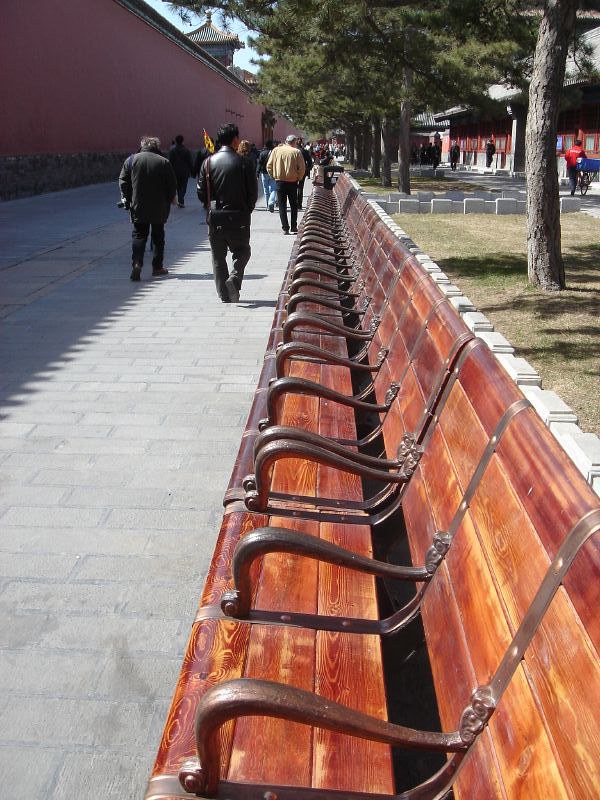The image captures a scenic park walkway lined with rows of connected benches. Each bench is comprised of individual seats made from rich, glossy mahogany wood with three upper slats forming the seat and four slats for the backrest. These seats are separated by brownish bronze metal armrests. The pathway in front of the benches is a gray, brick-like cement sidewalk, where four individuals are walking away into the distance—one in a black leather jacket, another in a plain black jacket, and a man in a tan jacket. The walkway is flanked by a plot of grass and a row of trees, adding to the scene’s natural beauty. Behind the benches, there is a white concrete barrier resembling a fence. The setting is completed with a tree full of leaves, and a brick building visible on the left. In the far background, the traditional roof of a building suggests an Asian architectural influence. The orderly rows of benches and the serene park ambiance form the primarily featured elements of this well-composed photograph.